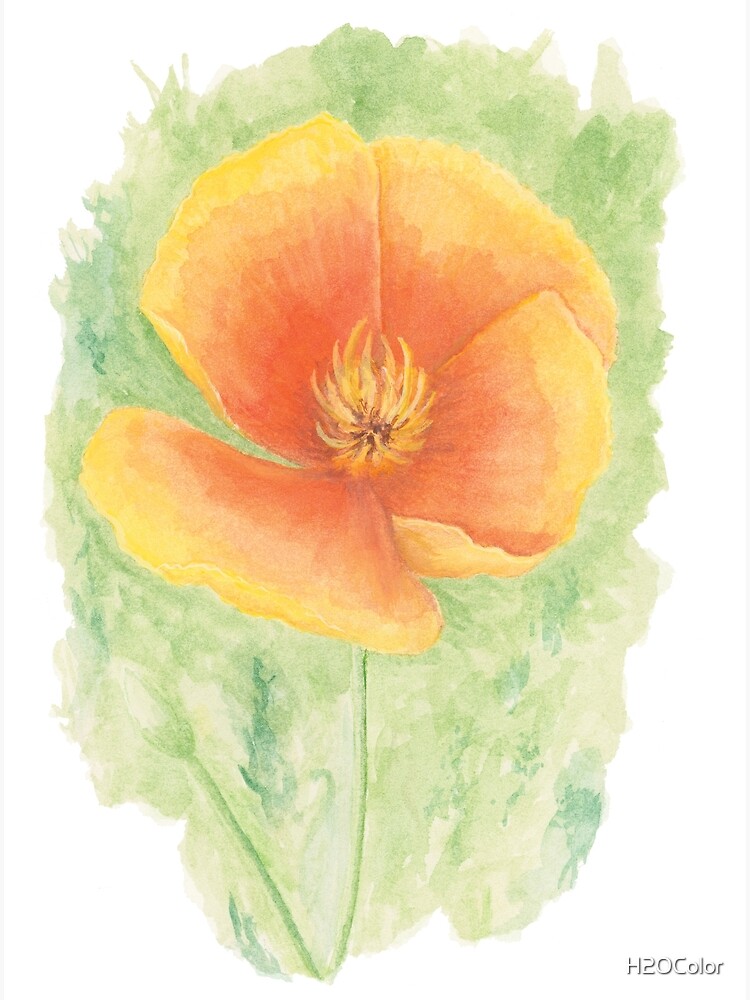This artwork is a vibrant watercolor painting of a flower, likely a hibiscus or a poppy, prominently featuring an open, orange blossom. The flower, displaying four large, radiant petals in varying shades from reddish-orange to bright peach, sits atop a green stem which extends upward. The petals are adorned with delicate, feather-like pollen filaments in the center, appearing in a mix of hay and peach colors. The background is a watery blend of green hues, transitioning from a deeper green at the top to lighter shades towards the bottom, with multiple stems emerging from the base. One of the stems supports an unopened bud, complementing the main bloom. The entire scene is framed with a white border, and at the bottom right, the text "H2O color" is subtly inscribed, emphasizing the watercolor medium.